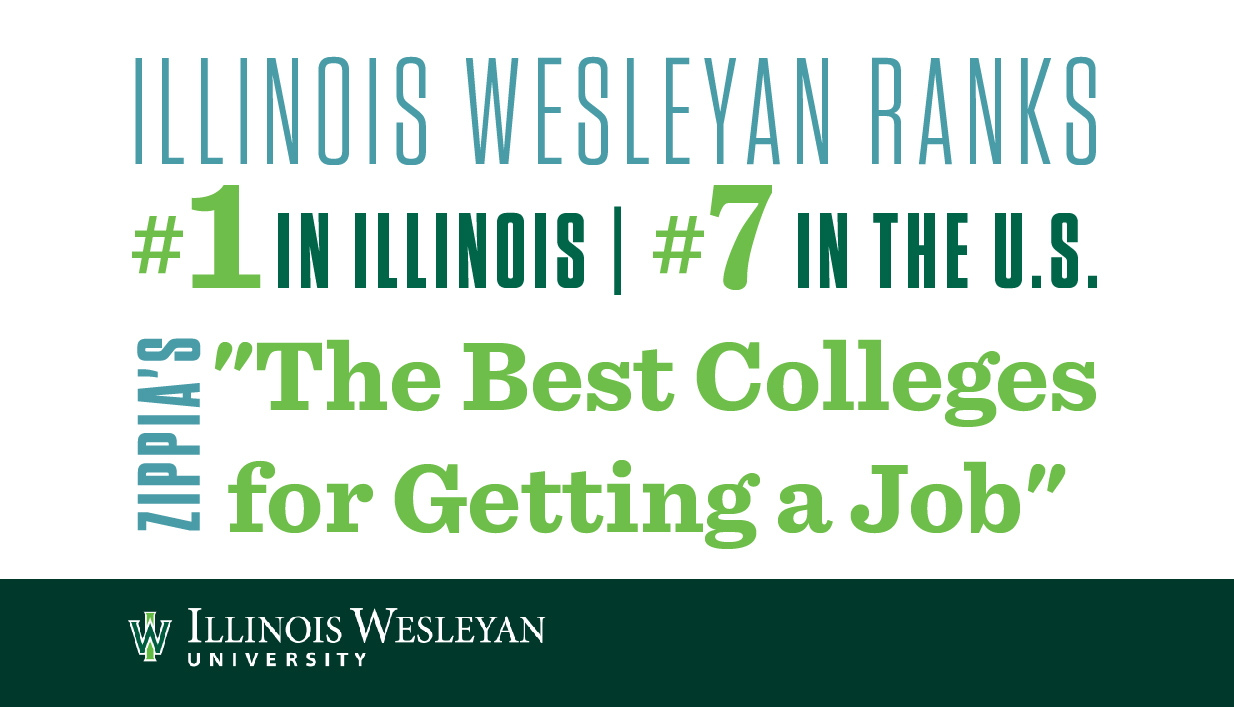The image appears to be a promotional advertisement, utilizing a striking combination of teal, forest green, and neon green fonts. The text prominently features the statement: "Illinois Wesleyan ranks number one in Illinois, number seven in the U.S., Zippia," highlighting the institution's prestigious standing. This is followed by a quote: "The best colleges for getting a job," also in vibrant neon green font.

Below the main text, a hunter green banner stretches across the image, displaying "Illinois Wesleyan University" in large, bold, white lettering. An additional design element includes a neon green line intersecting a forest green 'W,' emphasizing the university’s branding. 

The use of color, particularly the bold neon greens and the coordinated green tones, effectively captures attention and draws the viewer’s eye. All text, including the capitalized "I" in Illinois, "W" in Wesleyan, and "R" in ranks, is clear and easy to read, with the exception of a slightly blurry "7" at the bottom, which remains legible.

The composition is clean and uncluttered, focusing solely on the textual elements and ensuring the message is immediately clear. This visually appealing approach enhances the advertisement’s impact and readability.